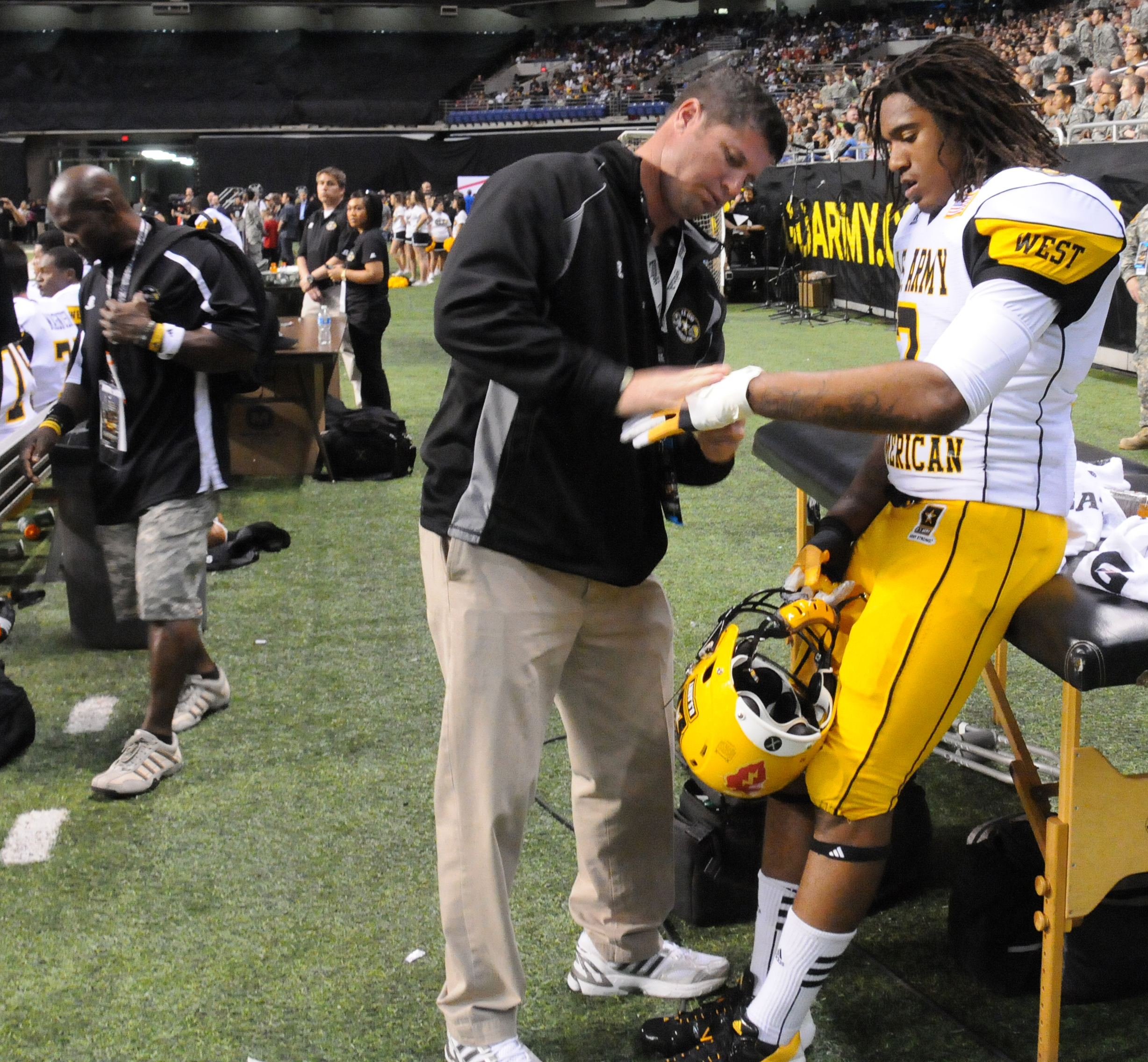The photograph captures a bustling scene on a green football field during a professional game, accentuated by a sea of spectators visible in the background. In the foreground, a Black football player, identifiable by his long dreadlocks, is being attended to by a White man who appears to be a doctor. The player, who looks to be in his 20s or 30s, is wearing a white jersey with 'Army West' partially visible on the front, hinting at 'West US Army' as part of the team's name. His uniform includes yellow shorts, and he holds a yellow helmet in his hand. He is seated and leaning against a portable black massage table with a wooden frame, positioned near the sidelines where cheerleaders and other players are also present. The physician, dressed in a black jacket, chino pants, and white shoes, concentrates on wrapping or massaging the player's hand. This scene is detailed with photographers and other onlookers milling about, capturing the intensity and urgency of the moment.